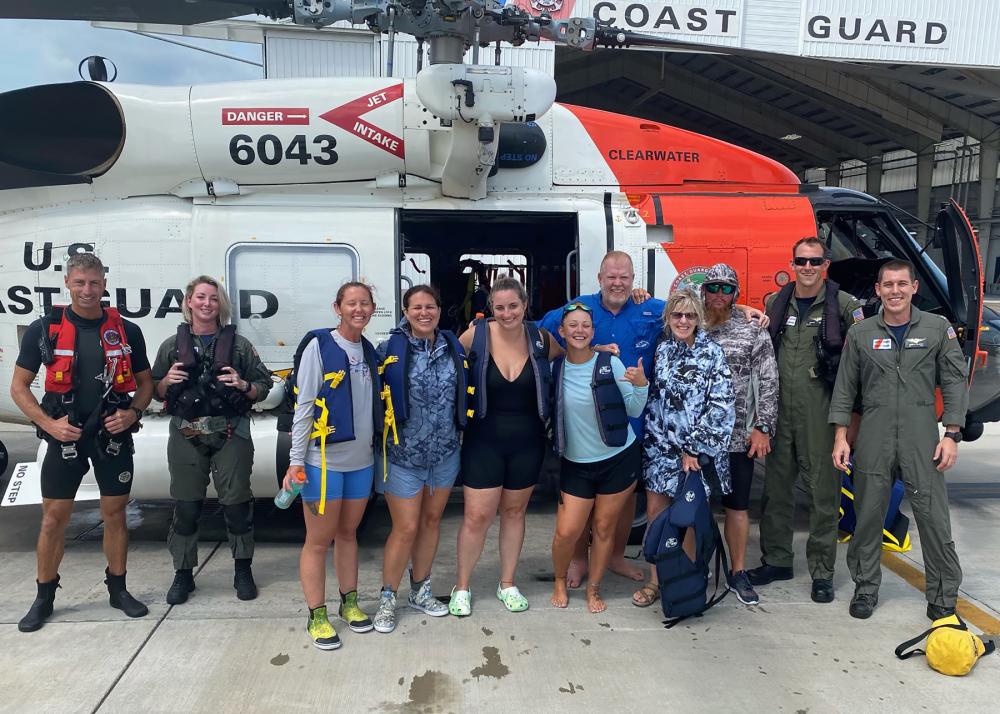The photograph showcases a group of eleven people posing in front of a U.S. Coast Guard helicopter. The helicopter, partly visible, has an orange front and a white body with "CLEARWATER" in black capital letters at the top. Prominently displayed on the side are the words "U.S. Coast Guard" and the identifier "6043" beneath warnings "DANGER" and "JET INTAKE." Some of the people are in Coast Guard uniforms; notably, a muscular man on the far left wears black biking shorts with a red vest, and two men on the right are in jumpsuits. Others are dressed casually, suggesting they might be friends or tourists. They stand on a concrete surface that shows brown stains. In the background, a white metal building with "Coast Guard" clearly visible on the front and a structure resembling a bridge can be seen. Additionally, a yellow bag is on the ground near the group.